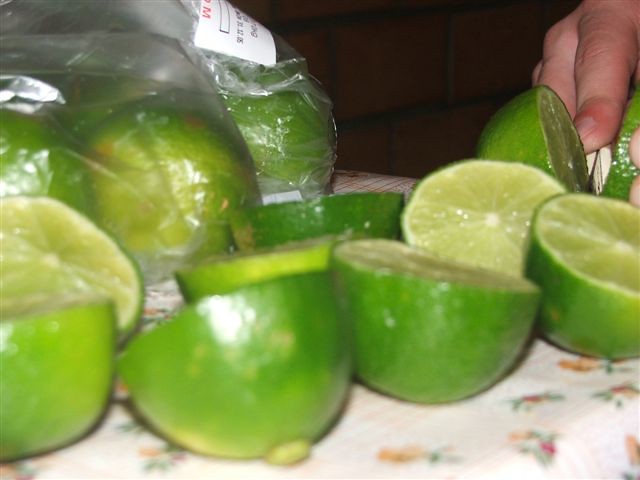This close-up digital photograph captures the intricate action of limes being sliced on a table. The image shows a variety of green limes, both whole and halved, arranged on a white tablecloth adorned with a floral design in orange, pink, and green. In the foreground, four limes are lined up, with three more behind them, two of which are tilted to reveal their lighter green flesh. In the upper left-hand corner, a partially visible clear plastic bag holds additional limes, marked by a white rectangular sticker with black and some red writing. Dominating the upper right corner, a slightly blurred hand, with the finger tip appearing red as if injured, is actively cutting through a lime with a silver knife. The person’s skin is light to medium in tone. The background is notably dark, with hints of deep brown bricks faintly visible, adding contrast to the scene.